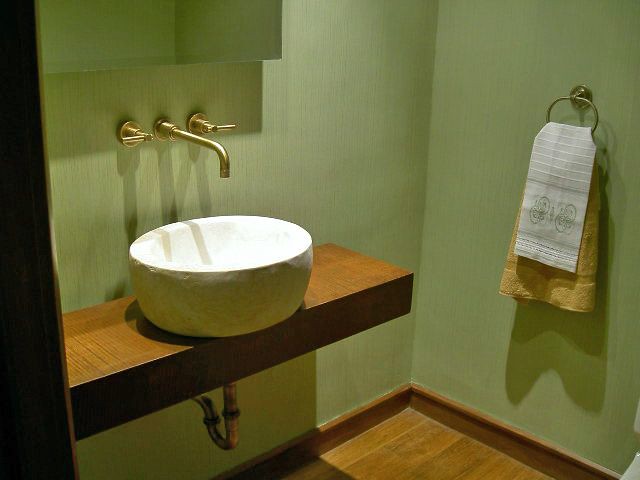The image depicts a bathroom with a rustic, wooden theme, featuring a wall-mounted vanity crafted from the same wood as the flooring. Atop the vanity rests a white vessel sink, which shows signs of wear with visible chips and damage. The plumbing beneath the sink is exposed, revealing a corroded and damaged metal structure. A pair of brushed chrome, wall-mounted faucets are installed in a spread mount configuration. An elongated faucet extends downward to fill the vessel sink, accompanied by two lever-style handles.

Above the faucets, a handle-less cabinet is mounted on the sage green walls, which display signs of wear and require cleaning. On the right-hand side, both the back and side walls are visible, adorned with a towel ring holding two towels. The front towel is a white hand towel with horizontal embroidered detailing, while a larger, yellowish bath towel hangs behind it. The towels cast distinct shadows on the wall due to the focused lighting in the room.

The hardwood floor matches the vanity, contributing to the cohesive aesthetic of the bathroom. Simple two-inch wooden baseboards line the bottom of the walls. The overall lighting is concentrated on the vessel sink, creating reflected highlights on the chrome faucets and casting direct shadows below.